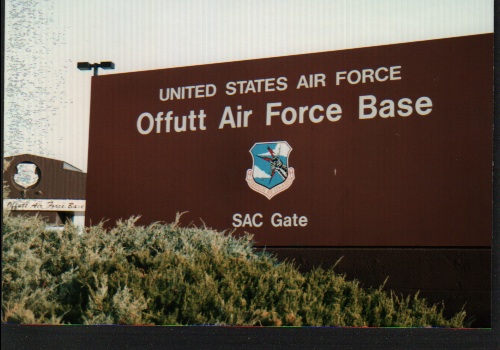This image is a grainy, rectangular photograph, likely taken with an older camera. It prominently features a large, rusty brown sign with the text "United States Air Force" in white, followed by "Offutt Air Force Base." Below this, there's a coat of arms symbol adorned with blue, white, black, and red colors, featuring what appears to be an aircraft. Beneath the emblem, in smaller white capital letters, it reads "SAC GATE." 

In the foreground, the bottom left corner of the sign is partially obscured by a grassy hill. There are shrubs in varying stages of decay, suggesting it is late in the season, with some areas turning yellow. To the left of the sign, in the background, the roof of a rounded, barn-like hangar is visible, although the writing on it is indistinguishable due to the distance and quality of the photograph.